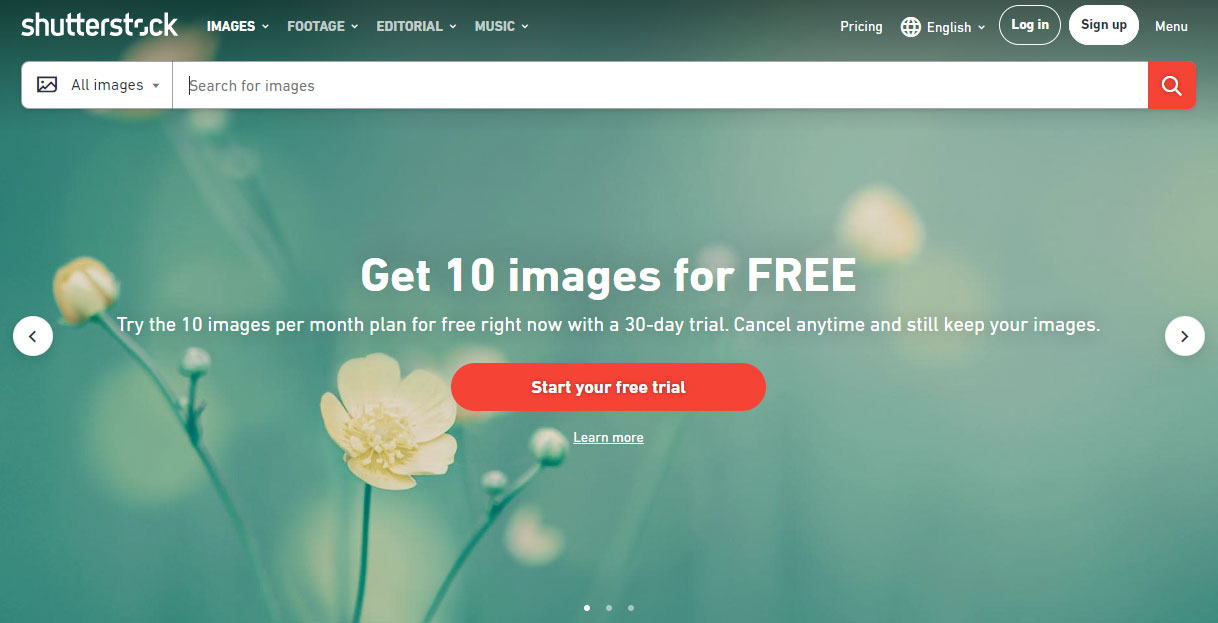This is a screenshot of the Shutterstock homepage displayed on a desktop computer. The background features a visually appealing gradient with different shades of green and teal. Towards the left, a yellow flower is prominently in focus, while additional petals and flowers blur into the background, creating a soft, blended effect.

At the top left corner, 'Shutterstock' is displayed in white text. To the right of the name, the menu bar includes several options: 'Images,' 'Footage,' 'Editorial,' and 'Music,' each accompanied by a small triangle to indicate a drop-down menu with more selections. Further right, the menu includes 'Pricing,' 'English' (with a drop-down for language selection), a circular button with a white background and bold white text labeled 'Login,' and a contrasting button with a white background and transparent bold text labeled 'Sign Up.' To the right of these buttons, the word 'Menu' appears in white text.

Below the menu bar, a search bar allows users to search for various images. Directly below the search bar, a bold text announces an offer: 'Get 10 images for free,' followed by a descriptive line. A large red button with white text encourages users to 'Start Your Free Trial.'